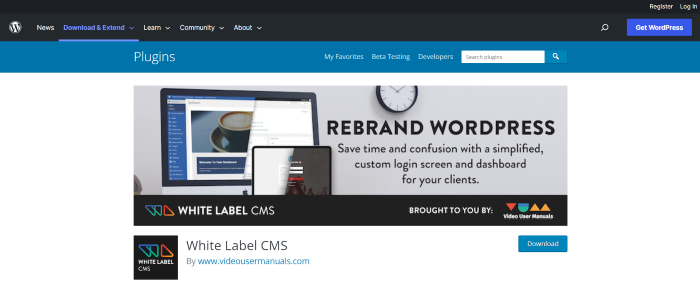This is a detailed caption for the provided image:

The image is a screenshot from a website interface. At the top, there is a black banner featuring a circular icon with a white background and a black capital "W" inside it. Adjacent to the icon is the word "News" in white text. Next in line are the words "Download" and "Extend," styled in a blue-purple font with a matching underline, accompanied by a down arrow indicating a drop-down menu.

Following these items in white text are the headers: "Learn," "Community," and "About," each with its drop-down menu. On the right side of the banner, the options "Register" and "Login" are visible, followed by a magnifying glass icon, suggesting a search function.

Beneath the top banner, there is a blue-purple tab labeled "Get WordPress," with "WordPress" written as a single word with a capital 'W' and 'P'. Below this is a teal-colored banner. Under the "Learn" section of this banner, "Plugins" is written in white text with a thinner font. To its right are additional options: "My Favorites," "Beta Testing," and "Developers."

Further down is a search bar with the placeholder text "Search Plugins" and a blue square with a white magnifying glass icon within it. The primary section of the page has a white background with a prominent banner stating, "Rebrand WordPress. Save time and confusion with a simplified custom login screen and dashboard for your clients."

At the bottom of the image is a black banner that reads, "White Label CMS. Brought to you by Video User Manuals." This is followed by the text, "White Label CMS by www.videousermanuals.com."